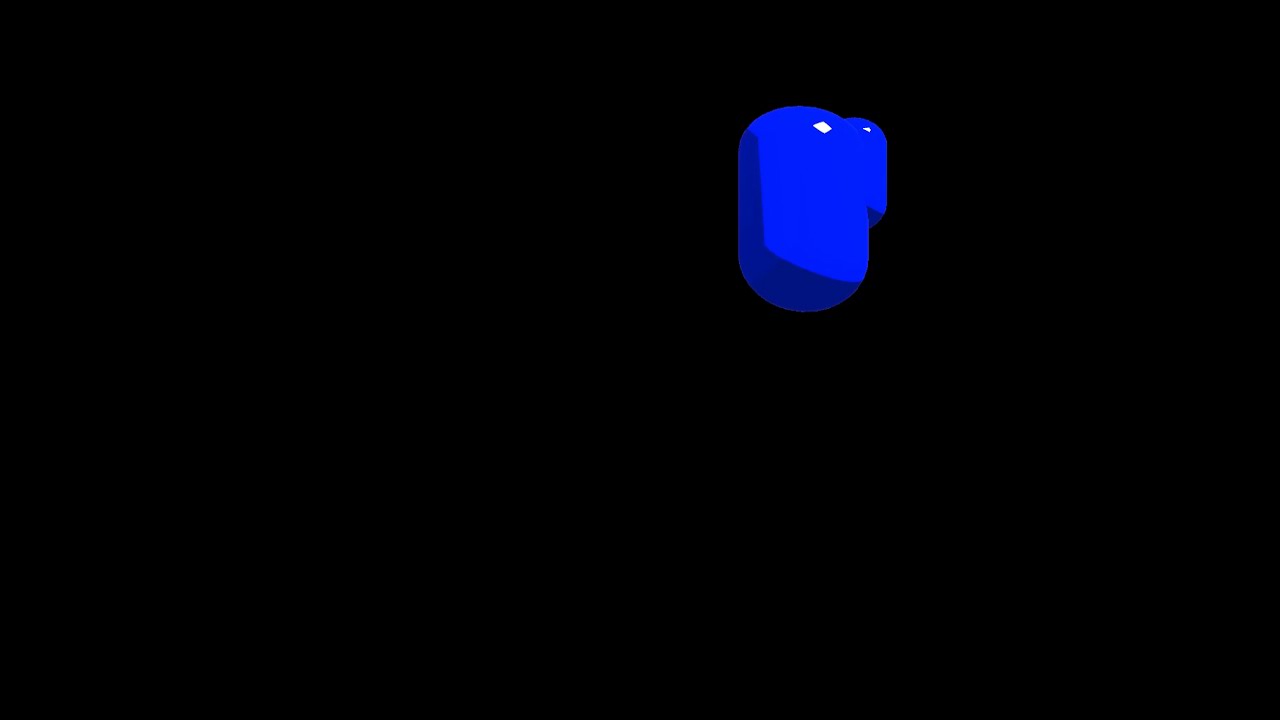In this horizontally aligned rectangular image, the predominant color is black, forming the background that swallowed almost all its space. Towards the upper right portion of the image, there's a small, three-dimensional, cylindrical blue figure that resembles a pill. Slightly behind this primary cylinder is a second, smaller blue cylindrical figure, barely visible, creating a layered effect. Both forms are distinctly painted blue, transitioning into a darker blue at the bottom. They feature tiny white spots: the main cylinder showcases a very small diamond-shaped white spot at the top and a tiny triangular white spot to the right. The contrasting flat black backdrop and minimalistic blue shapes give an isolated, almost floating impression, occupying roughly 10% of the entire image, emphasizing their diminutive presence against the vast empty space.